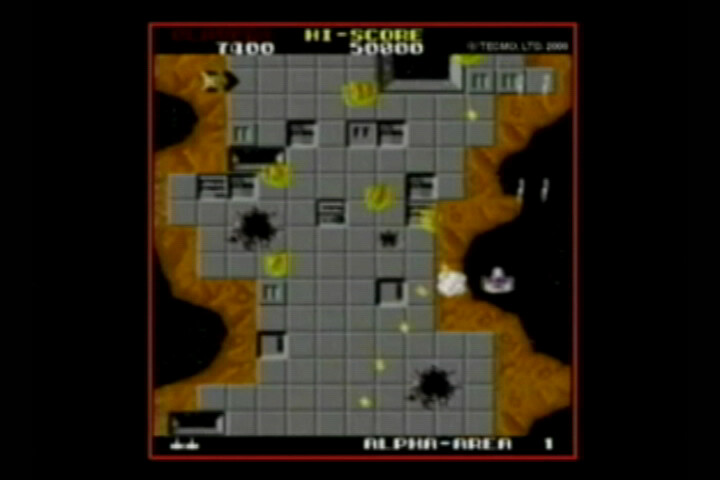This image captures a somewhat blurry screenshot of a video game displayed on a screen. The game's backdrop is entirely black, dominated by a thin red square outline that frames the main playing area. Inside this red square lies an irregular gray shape composed of numerous smaller gray square tiles, suggestively akin to a bombed or damaged grid, with some black holes punctuating the tiles as if by explosions. Interspersed amongst these tiles are yellow blobs, reminiscent of fire or explosions, and splashes of orange-red color accent the outer edges of the gray squares, enhancing the visually chaotic scene.

At the top of the image, the text "HIGH SCORE" is prominently displayed in yellow, with two sets of scores below it in white: 50,800 and either 400 or 1,400, as the exact number is unclear due to the blurriness. The background also hints at organic elements, with the gray grid seemingly superimposed over a brown landmass-like shape. Towards the bottom of the screen, the text "alpha-area 1" can be discerned, albeit somewhat blurred, suggesting a level designation. Additionally, there are small icons in the bottom left corner that possibly indicate remaining lives, providing further insight into the gameplay mechanics.